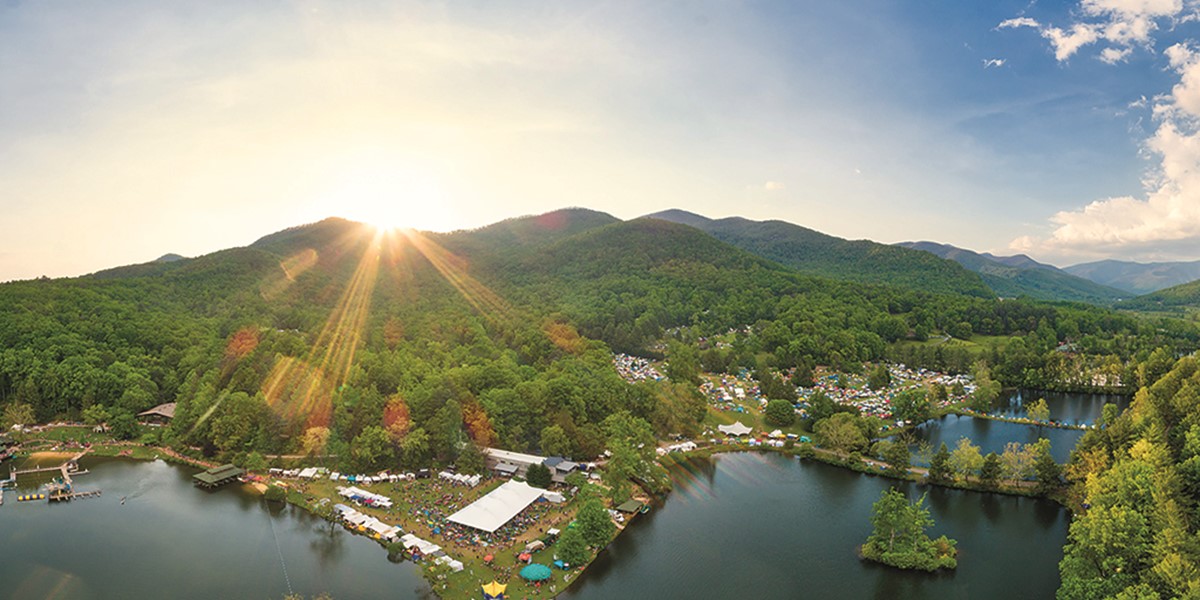This aerial photograph captures a lakeside scene where a vibrant festival appears to be taking place. The image, likely taken during summertime, offers an expansive view of tree-covered mountain ranges that stretch into the distance over the horizon. Numerous large tents and festival-type awnings are set up along the beach, clustered at the water's edge, and are surrounded by many people partaking in the event. Some of these tents resemble camping structures, suggesting that attendees may be staying overnight. The clear blue sky indicates a sunny day, with the sun's rays casting a warm glow across the mountains and treetops, hinting at late afternoon. The lake's calm, dark waters feature a boating dock on the far left, where a single boat is moored close to a small pavilion or boathouse that extends into the water. Overall, the lively atmosphere, combined with natural beauty, promises an enjoyable event amidst picturesque surroundings.